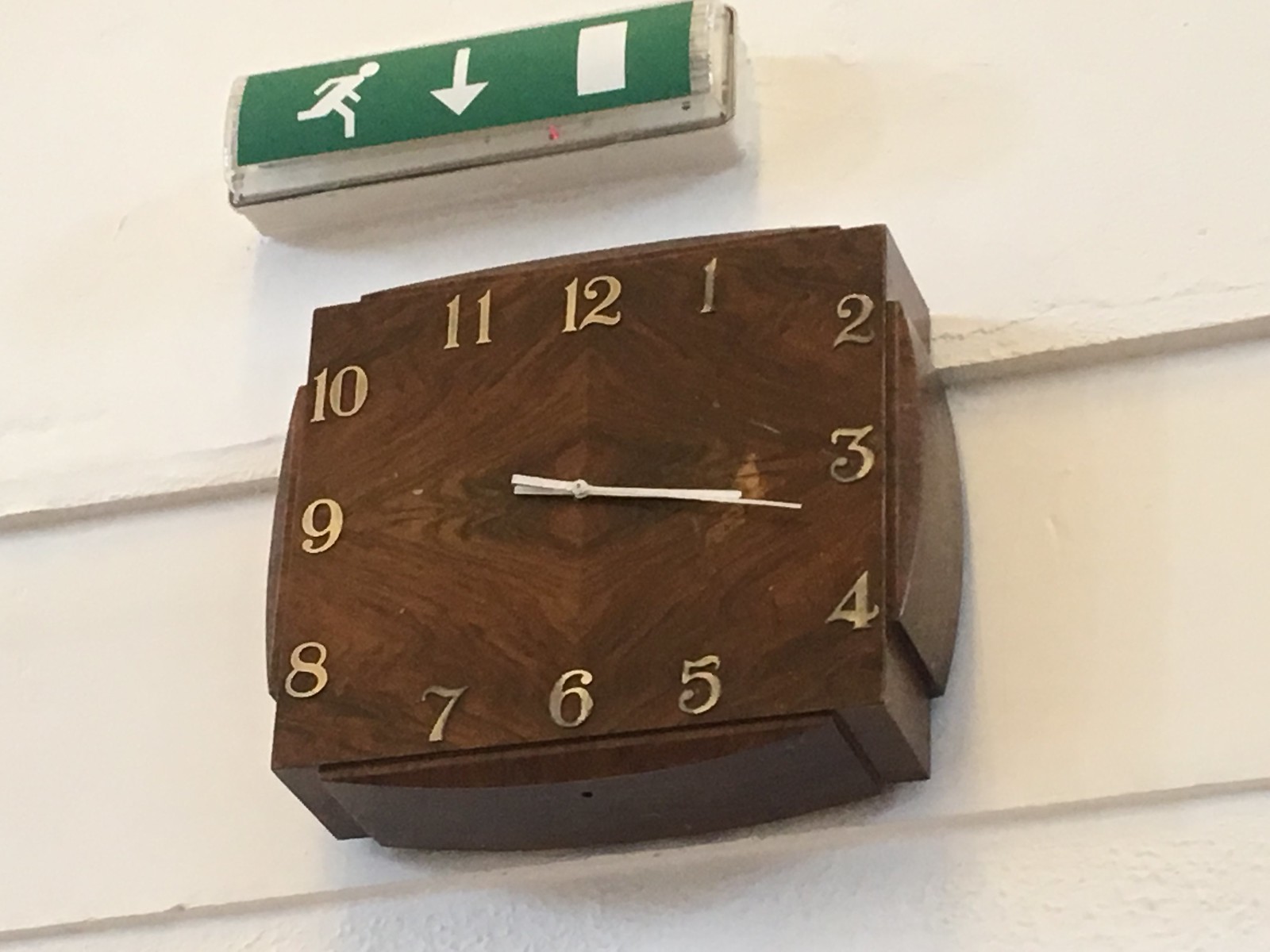This image is a photograph depicting a section of an interior space with a white wooden wall, divided into long panels segmented by horizontal wooden borders. At the top of the wall hangs a green sign featuring a series of white symbols: a running stick figure, a downward-pointing arrow, and a small vertical rectangle, possibly indicating an exit or elevator. Directly below this sign is a square-shaped analog clock, crafted from what appears to be a chunk of wood. The clock face features gold numbers from 1 to 12, with white hands indicating the time as 3:17.